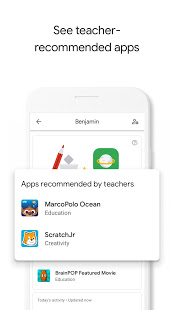In the screen capture, at the top, the header displays the name "Benjamin" with a left arrow pointing towards the left and an icon on the right side. Below, there's an icon of a red-colored pencil and paper. Adjacent to it, there's a green button featuring a stylized image of a ringed planet, resembling Saturn, with a yellow ring around a white planet.

Overlaid on this section is a panel titled "Apps Recommended by Teachers." The first app featured is "Marco Polo Ocean," represented by an icon of an animal with brown skin, white round eyes with black pupils, and brown fur, labeled as educational. The second app is "Scratch Junior," illustrated with a tiger that has an orange face, white muzzle, and a black nose, labeled as fostering creativity.

Returning to the screen, still overlaid by the pop-up, it mentions "BrainPOP Featured Movie," tagged as educational. This is depicted by an image resembling the Sun: a brown central circle with white eyes, surrounded by alternating dark blue and light blue rays. At the very bottom, there are some blurry letters that are difficult to read.